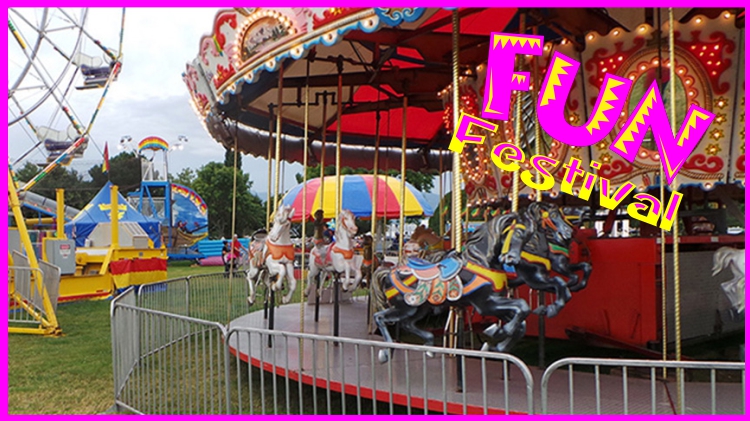This vibrant and colorful photograph captures the lively atmosphere of a carnival. Dominating the foreground is an illuminated carousel, encircled by a metal fence. The carousel is adorned with intricately detailed horses, the two prominent ones being black with yellow, red, and blue ornate saddles, while more white horses with similarly elaborate designs are visible in the background. Radiant lights enhance the carousel's festive aura. Just behind it and to the left, a Ferris wheel looms, partially visible and contributing to the scene's overall charm. Further back, an exuberant array of tents and additional rides punctuate the scene, with a canopy featuring a striking pattern of blue, red, and yellow. One tent has a traditional pointed top, and a possible pirate ship ride can be glimpsed in the distance. Overlaid in a playful purple and yellow spiky font, the words "FUN" and "Festival" appear, with "FUN" in giant uppercase letters and "Festival" in smaller, capitalized below. The text is positioned at a jaunty angle on the upper right-hand corner, framed by a purple border that completes the festive look. The overall color palette of red, blue, and yellow resonates throughout the image, encapsulating the carnival's exuberant spirit.